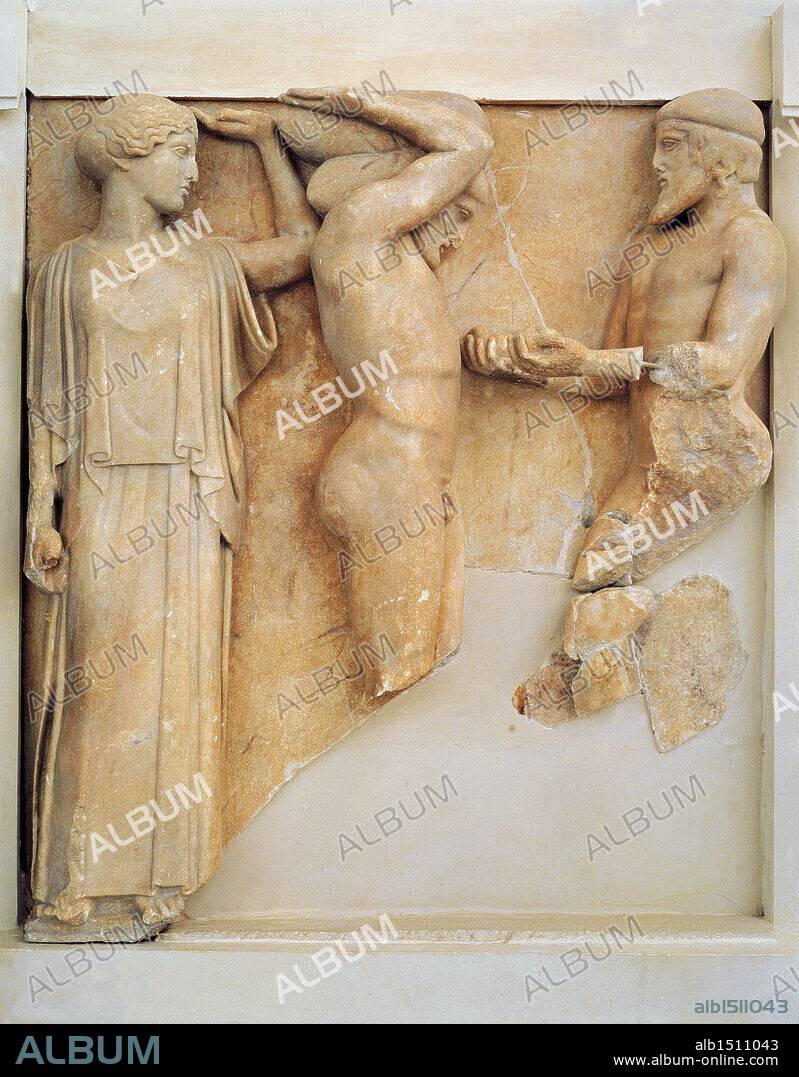The image is a vertically rectangular photograph of a frieze depicting three carved human statues against a cement background. Stamped repeatedly across the image is the word "album" in varying colors, with a black band at the bottom displaying the word "album" in blue or gray letters. Numbers are also present along the side, alongside a URL, www.albumonline.com, in the lower right corner, indicating the image's creator.

On the left is a female figure with her left hand raised toward the ceiling. Positioned next to her is a middle figure, a man dressed in a long, flowing tunic, with his left hand also extended upwards, palm facing the sky. The middle figure appears to be naked and is carrying what looks like bundles of burlap sacks on his shoulders. On the right, there is another male figure with his hands extended, appearing to receive the sacks. This figure wears a small cap, has a beard, and short hair. Notably, the statues on the right and in the middle are fragmented and partially broken, suggesting they might be in the process of reconstruction.